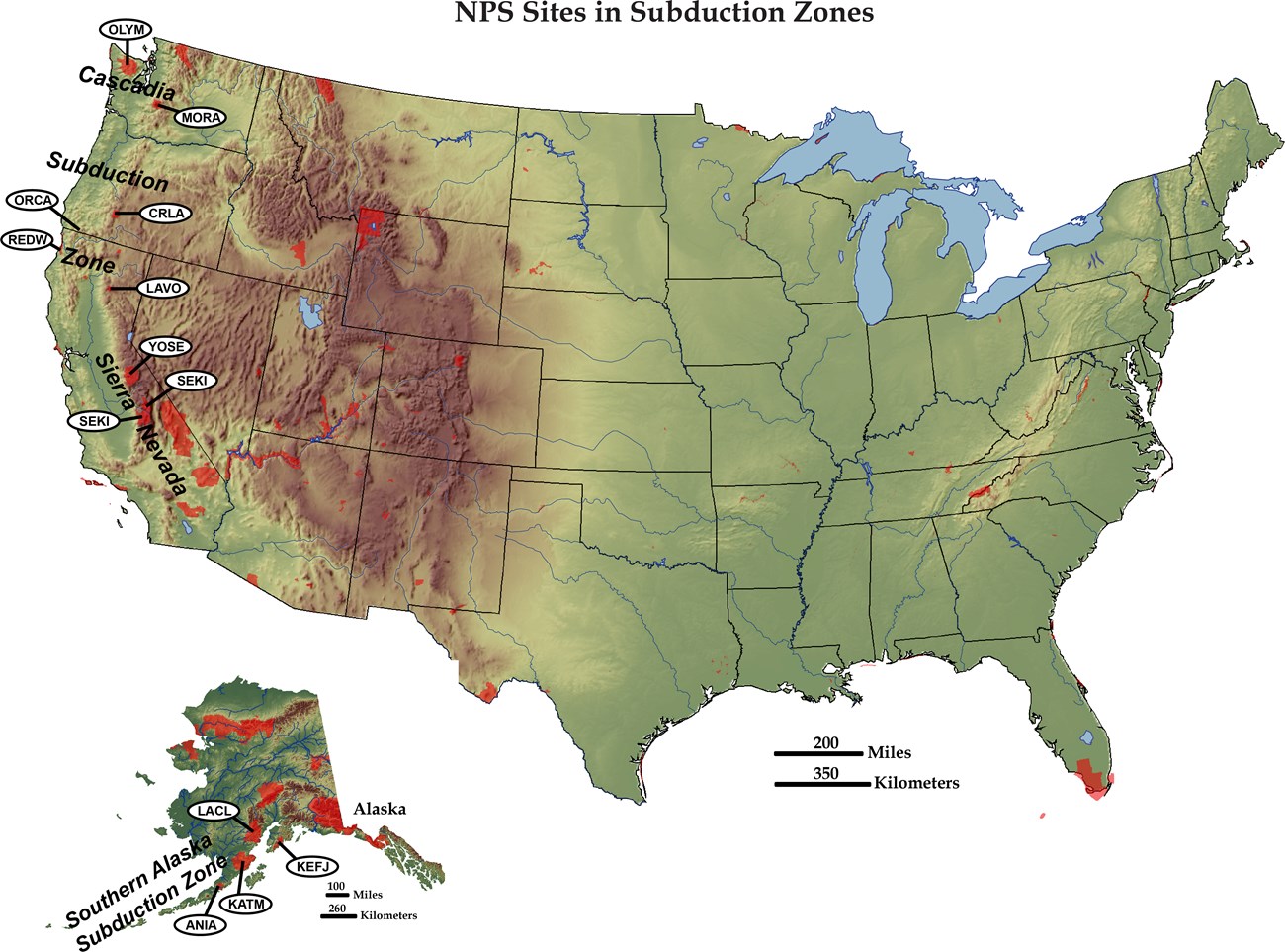This detailed topographic map of the United States, including a separate inset for Alaska in the lower left, highlights National Park Service (NPS) sites in subduction zones. The map primarily uses shades of green to represent different land terrains, with browns indicating mountainous regions, particularly in the western areas around Nevada and California. The top of the map prominently displays "NPS sites in subduction zones" in black. Various labels across the map identify significant subduction-related features: the Cascadia subduction zone near Washington state, the Sierra Nevada in California, and the southern Alaska subduction zone. Red spots and white ovals with four-letter codes mark specific NPS sites within these zones. A legend in the corner provides scales in miles and kilometers, though the map lacks a detailed explanatory legend for the color coding.